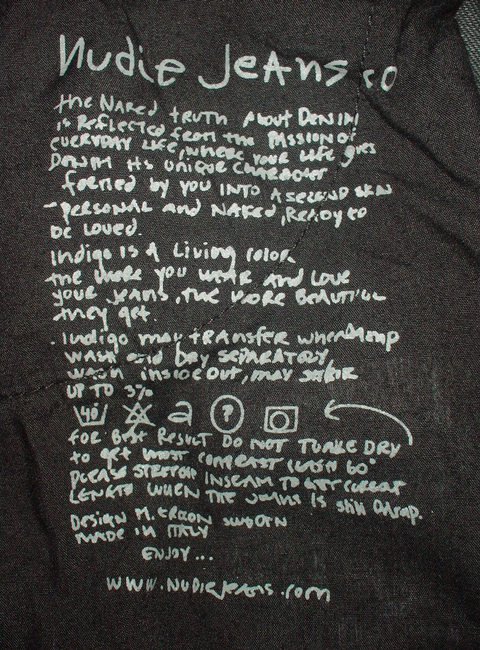This black and white photograph features a detailed close-up of a clothing label, likely from a t-shirt made out of a soft, slightly crumpled fabric. The label is prominently marked with the brand name "Nudie Jeans, CEO" at the top in bold white lettering. The majority of the label is densely packed with small, handwritten text, creating a textured visual effect. While most of this text is difficult to decipher, phrases such as "indigo is a living colour" can be discerned. Towards the bottom of the label, a series of washing symbols is present, accompanied by an arrow, suggesting the presence of washing instructions that are challenging to read due to their small size. The label concludes with the brand's website, "www.nudiejeans.com," also in white lettering, providing a clearer point of reference amidst the intricate design of the label.